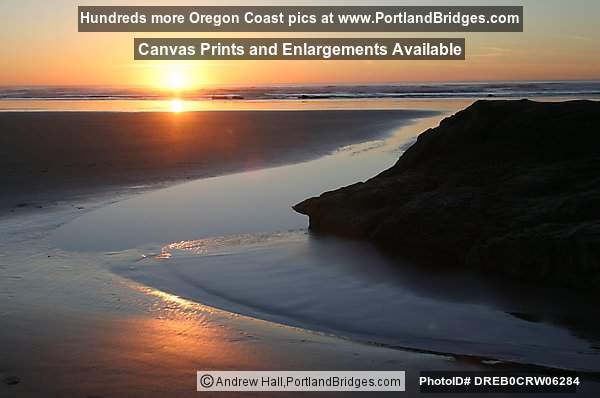This is an aerial, angled view of the picturesque Oregon coast at sunset. Dominating the right side of the image is a large, rocky hill, whose silhouette adds dramatic contrast to the scene. At its base, white sands stretch out to meet the ocean, their surface gleaming with reflections from the setting sun. The entire atmosphere of the photo is bathed in rich, sunset hues of orange and green, with the glossy wet sand mirroring these colors. Above the scene, a black rectangular banner reads, "Hundreds More Oregon Coast Pics at www.portlandbridges.com," while a second black banner below it promotes, "Canvas Prints and Enlargements Available." Against the breathtaking backdrop of the sun dipping below the water, captured by photographer Andrew Hall, a white banner at the bottom center of the photo states, "Copyright Andrew Hall www.portlandbridges.com," with an additional black banner in the bottom right corner displaying the photo ID.